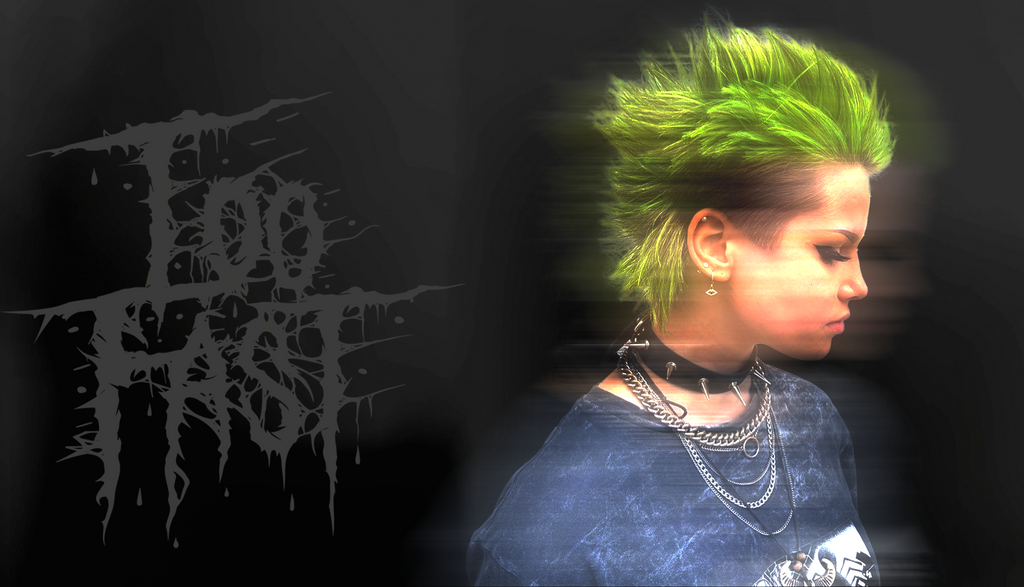The photograph features a young woman, likely in her late teens or early twenties, positioned on the right side against a completely black background. She embodies a punk rock or metal aesthetic with elements that cross into goth culture. Her hair is distinct: shaved on the sides and sporting a spiky green mohawk approximately three inches in length. Captured in profile, she gazes downward toward the lower right corner of the image, giving the impression of subtle movement as if she's walking away.

Her style is accentuated by multiple earrings in her right ear, a studded spike choker, and several silver-linked necklaces. Her eyeliner is thick, complementing her edgy look. She wears a navy blue band shirt, hinting at her musical preferences. The words "too fast" are emblazoned to her left in a graffiti-like, barbed-wire font that appears slightly blurred, enhancing the sense of motion and chaos. The combined elements create a vivid, rebellious image that straddles punk rock and goth influences.